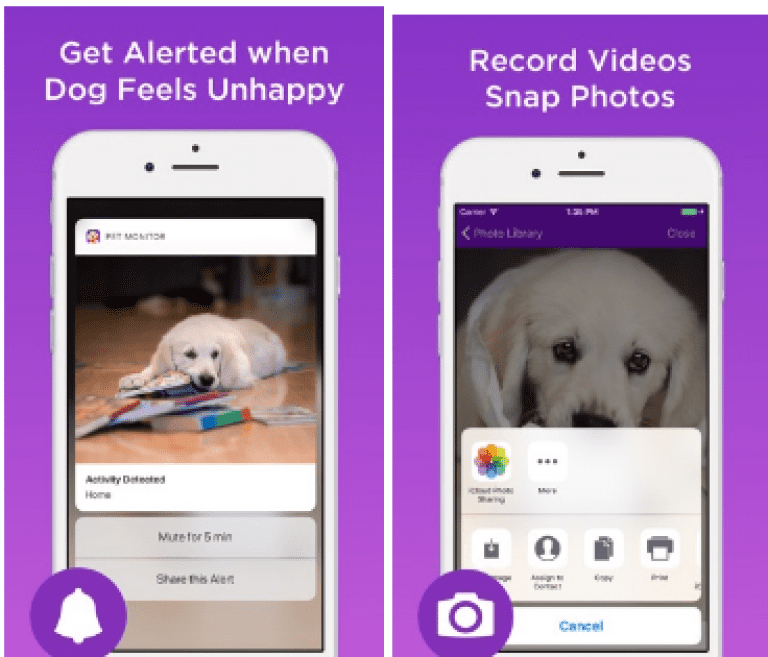Here is a more polished and detailed caption for the described image:

"In this composite image featuring two smartphone screenshots set against a purple background, the focus is on a pet monitoring app. Above the left phone, white text reads 'Get alerted when your dog feels unhappy.' The phone screen displays an alert indicating that a white dog has been 'actively detected at home,' with an option to 'mute for 5 minutes' underneath the dog's image. The right phone screenshot has white text above it that says 'Record videos, snap photos.' This screen also features an image of the same white dog. Both phones highlight the app's ability to monitor and interact with pets, with clear instructions and visual aids to guide the user."